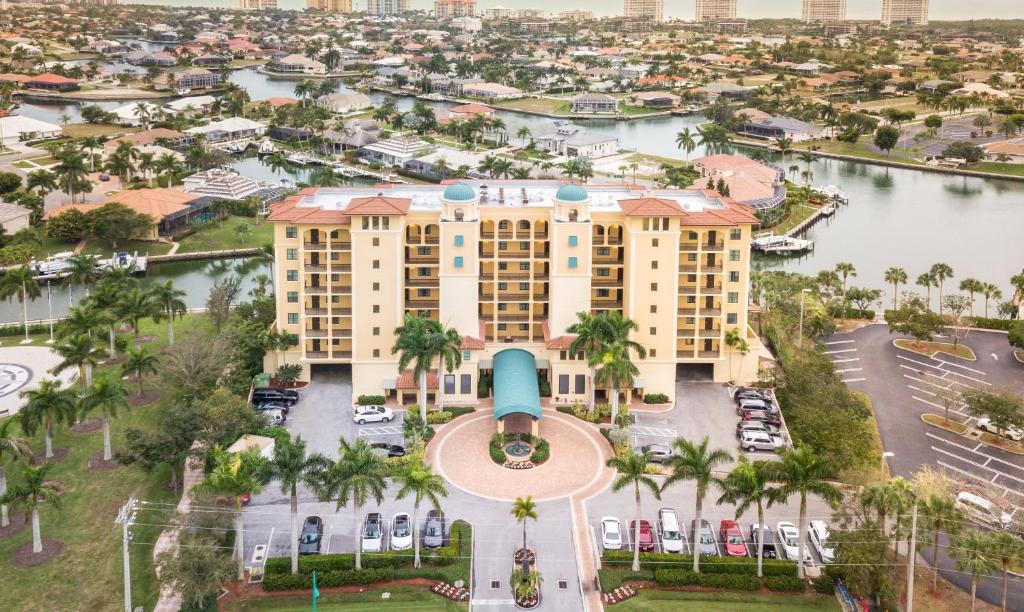The image is an aerial view looking down onto a large, six-story hotel, which serves as the focal point in the center of the photograph. The hotel is a beige color with pink accents on the roof and has a turquoise awning covering the entrance walkway. The hotel is surrounded by numerous palm trees and several cars are visible in the front parking areas, with additional parking to the right of the building. In front of the hotel is a circular driveway, creating a grand entrance. The background features an intercoastal area with water channels weaving through plots of land, which are dotted with houses and luxury homes. The surrounding landscape includes more palm trees, lush greenery, and other buildings, giving the impression of a resort-like, tropical environment. In the distant background, there are taller buildings, possibly hotels or skyscrapers, adding to the luxury coastal setting.